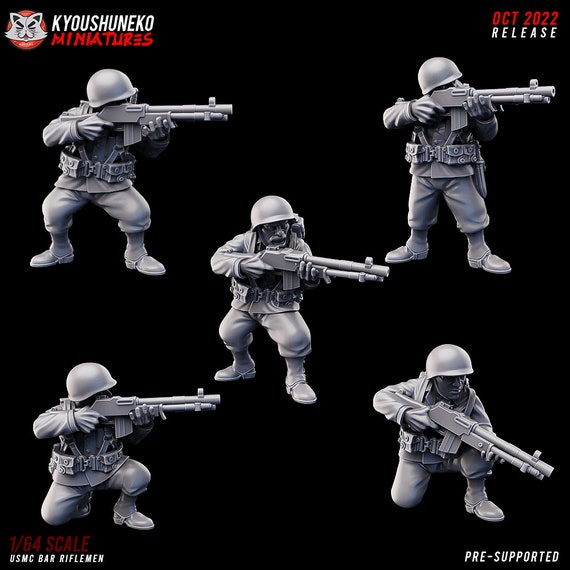This advertisement from Kaiyushuneko Miniatures features highly detailed 1:64 scale USMC Bar Riflemen miniatures set for release in October 2022. The ad showcases five different angles of the same soldier figurine, all of which are pre-supported for easy assembly and painting. The soldiers are depicted in various combat poses, including standing, kneeling, and aiming their rifles which resemble AR-15s. Each figurine is meticulously crafted with military uniforms, helmets, gun belts, and heavy boots, making them ideal for collectors and enthusiasts of military miniatures. The company's name, Kaiyushuneko Miniatures, is prominently displayed with a cartoon cat logo, and the ad features clear markers for "October 2022 Release" in red and white text.